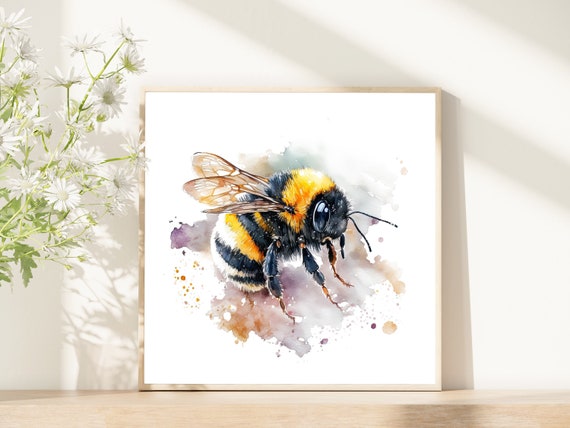This up-close photograph captures a detailed painting of a bumblebee on a large square canvas, roughly three feet by three feet. The canvas, which has a white background, is placed on a wooden table and leans against a white wall. The bumblebee, painted with intricate detail, features alternating black and yellow stripes along its short, stubby body. Its head is black with large black pupils, and it has two black antennae extending from its head. The bee's legs are primarily black, with one brown exception, and it possesses short, brownish-opaque wings situated mid-body. The painting employs shadowing around the bee's abdomen, head, and wings to create a nearly three-dimensional effect.

Surrounding the bee are small splotches of watercolor in hues of purple, orange, and beige, which enhance the contrast and make the bumblebee painting stand out. To the left of the canvas, there is a small potted plant with light green leaves and an abundance of delicate white flowers, casting a soft shadow on the wall in the well-lit indoor setting. Stark shadows of possibly diatom bars add a distinctive touch to the overall imagery, contributing to the room's bright and vivid atmosphere.